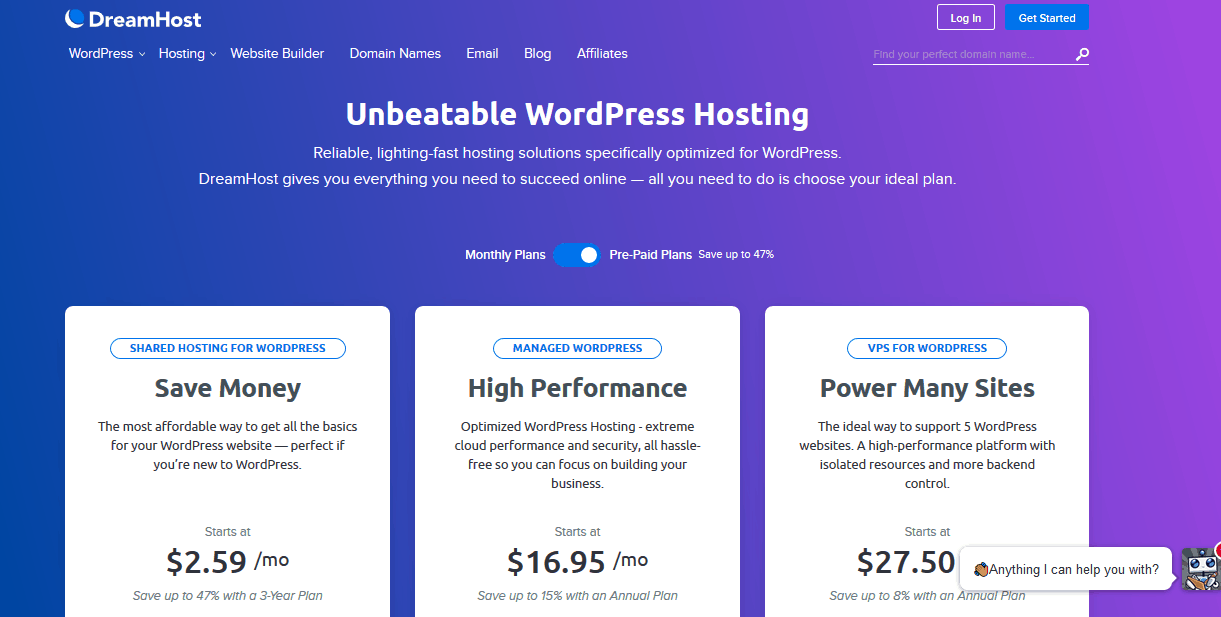The image features a promotional layout with multiple design elements and information points. In the top left corner, the word "Dreamhouse" is prominently displayed in white text, accompanied by a blue circle and a half-moon graphic. Below there are interactive buttons, with one labeled "Login" inside a rectangle and another saying "Get Started."

The main content sections covered are "WordPress Hosting," "Website Builder," "Domain Names," "Email," "Blog," and "Affiliates." The phrase "Unbeatable WordPress Hosting" is emphasized as a key selling point. Text claiming "Dreamhost gives you everything you need" suggests comprehensive service offerings, with a prompt to "add your plan."

Further details include a mention of "Monthly Plans" and the potential to "Save up to 47%," suggesting cost-saving benefits for users. The focus appears to be on shared hosting for WordPress, emphasizing affordability and basic features necessary for a WordPress website.

Additional text highlights the complexity of WordPress solutions and the ease provided by Dreamhost, implying a simplified hosting experience. Mentions of supporting Fiverr and the utility of hyperlinks for control in the background are also present, although their relevance to the main hosting offering is less clear.